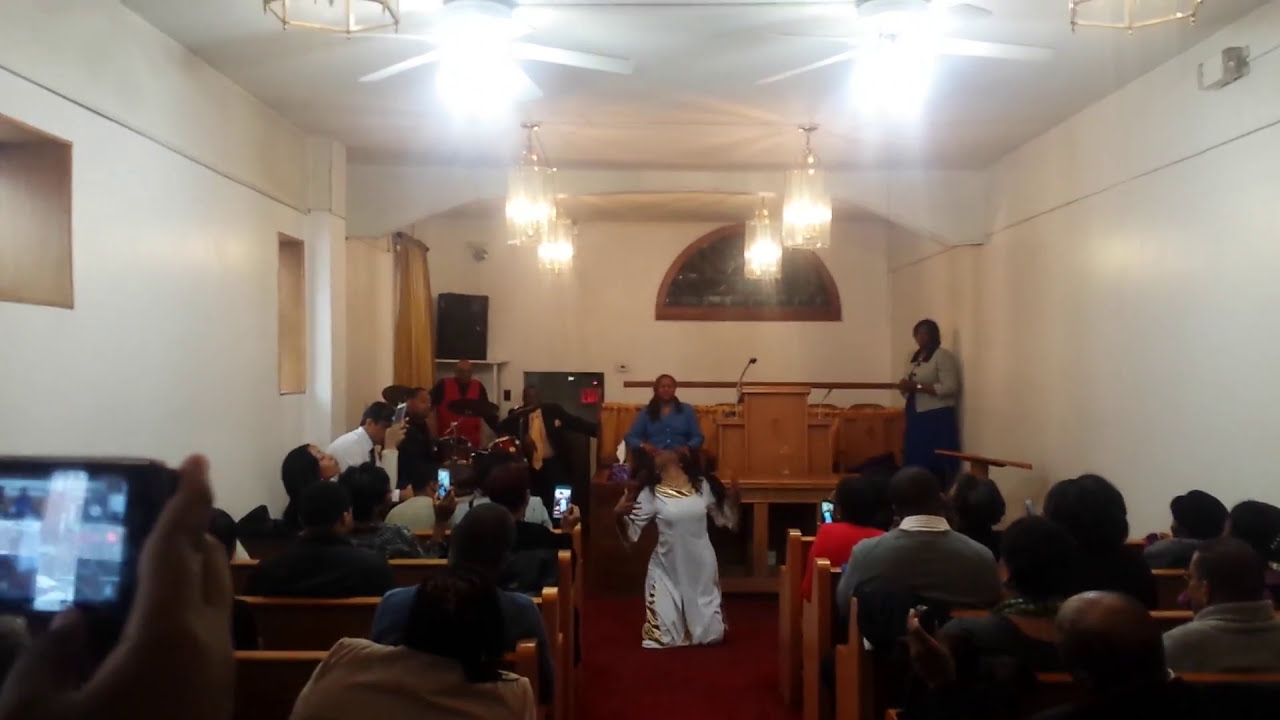The photograph captures the bustling interior of a small church, featuring white walls and a ceiling adorned with golden hanging lights and fans. The camera is positioned in the central aisle between wooden pews, which are filled with numerous engaged African American congregants. The focal point of the image is a significant healing or revival scene taking place in the front-middle aisle, where a woman in a blue shirt stands with her hands on the head of a kneeling woman in a white dress, who appears to be in a state of spiritual exaltation. Behind them, along the back wall, a musical band is actively playing, adding to the lively atmosphere. Several people in the pews are capturing the event on their smartphones, further highlighting the importance of this moment. Near the stage, framed by a large speaker and a curtain on the left, and a podium with mics on the right, the event appears to be set for a significant religious or dramatic performance.